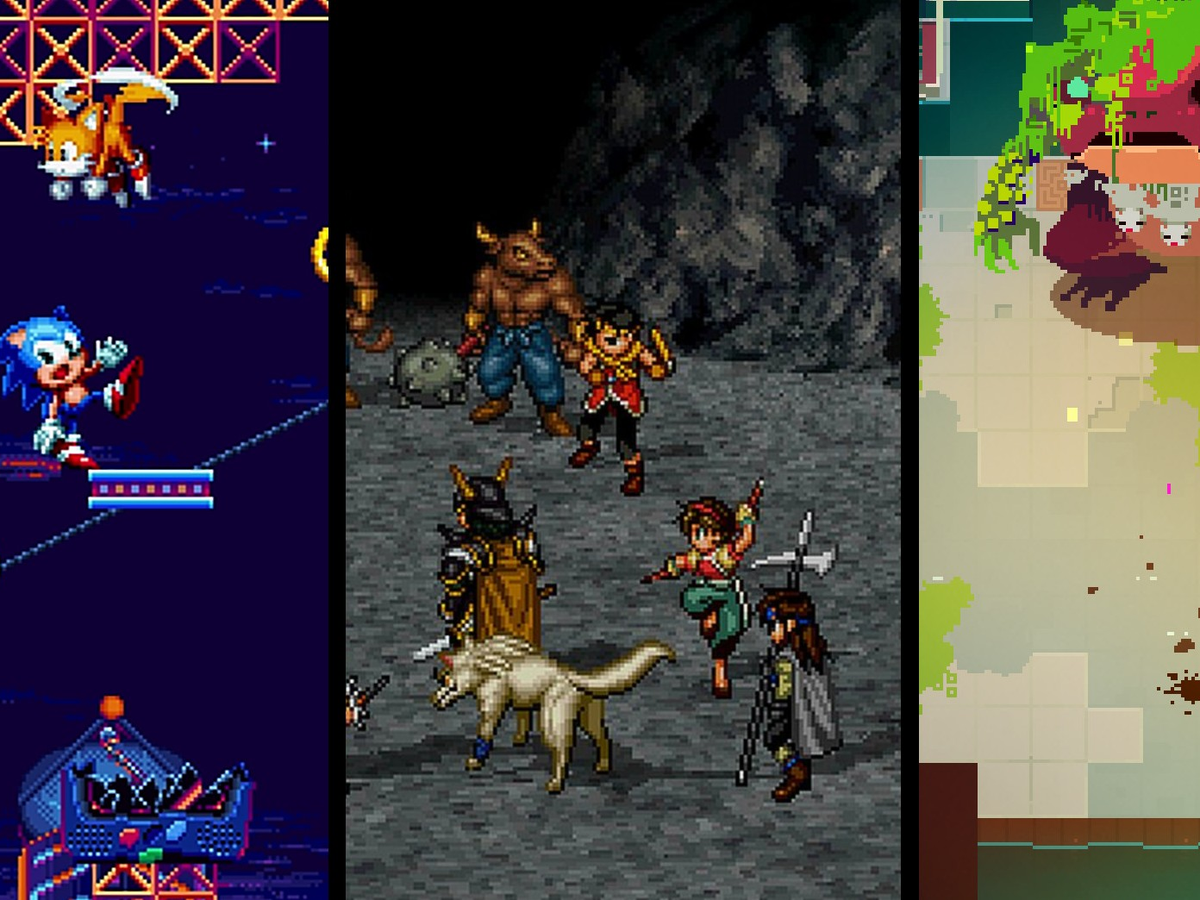The image is a composite of three separate video game scenes. On the left side, with a dark blue background, features characters from the Sonic the Hedgehog series. At the top, Tails, the fox with brown fur, white face, and gloves, is flying by twirling his tails. Below him, Sonic, the blue hedgehog, is standing with one foot and one hand in the air, seemingly about to move forward. There's an indistinct blue object at the bottom.

In the center, set in a cave-like gray environment, a minotaur-like creature wielding a spiked mace stands at the top. Below, a boy dressed in red with a bandana on his head is ready for combat. A girl in green pants and a battle pose is next, followed by a person with a large weapon and a cape. Additionally, there is a dog or wolf with a blue band around its leg.

On the right side, the scene shifts to another game with a predominantly green and soil-like surface. The details are less clear, but it includes undefined characters and elements with some red and brown tones at the bottom. Possibly, there's a creature that resembles a buffalo, but the specifics are hard to discern.